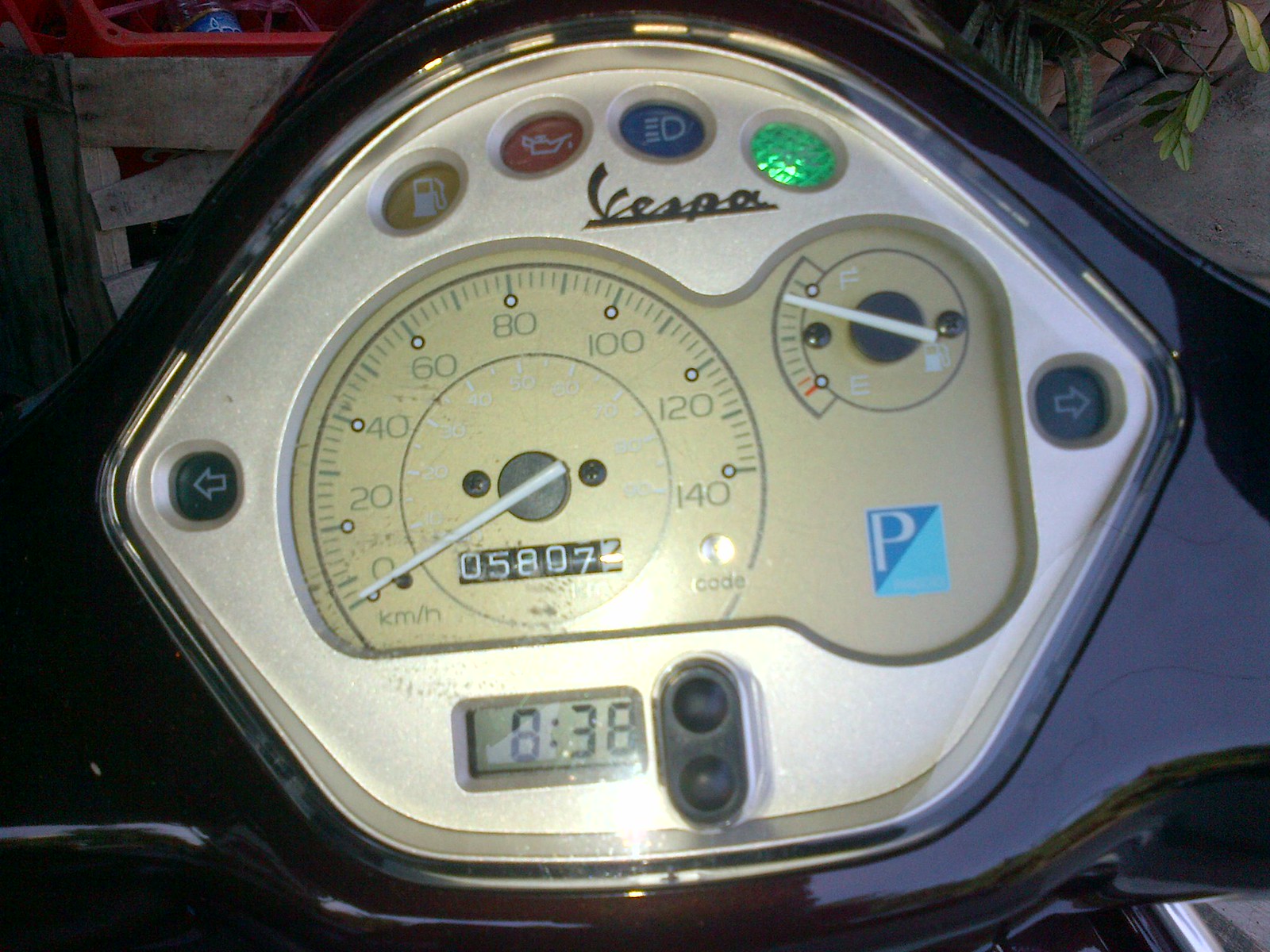This image displays the dashboard panel of a Vespa motorbike. Prominently at the top, the brand name "Vespa" is showcased. Below this branding, a digital clock reads "8:38." Flanking the sides are indicator lights, represented by small green dots. At the panel's bottom, black dots of some nature are present. The speedometer is centrally located, showing a current speed of 0 kilometers per hour with an incremental range from 0 to 140 km/h. The odometer reads "58,072" kilometers.

The fuel gauge, positioned at the lower section of the panel, indicates that the fuel level is nearly full. Various other warning and indicator lights are dotted around the panel – a green light is illuminated at the top right. Additional lights include an oil light (yellow), a gas light (yellow), and a high beam light (blue), with another oil light glowing red. 

The entire dashboard is set against a sleek silver panel with the outer edges framed in black. The background appears to be a shop, adding a contextual setting to the image.